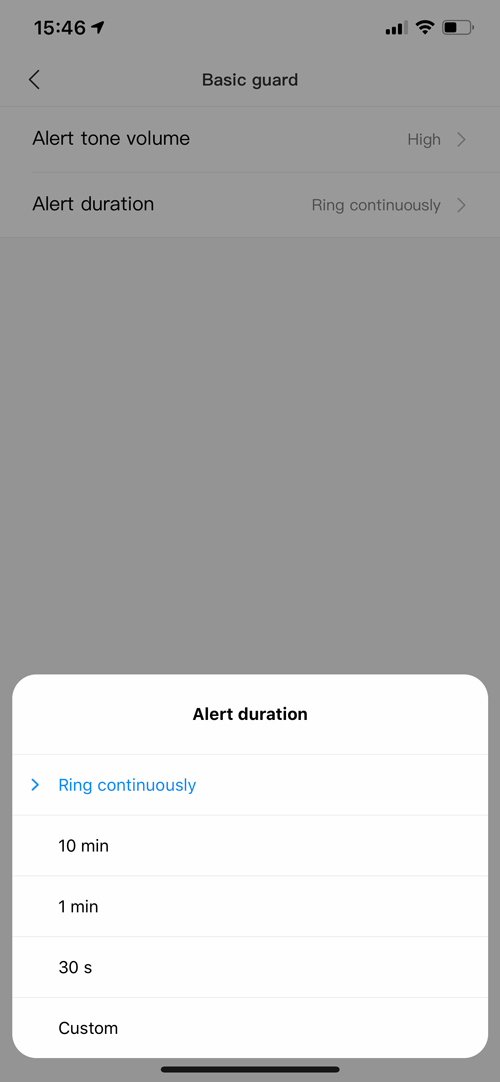**Detailed Caption:**

In this image, a user interface is displayed against a purple background. At the top of the interface, the number "1546" is prominently positioned with an upward-pointing arrow next to it. Following this is a leftward-pointing arrow accompanied by the phrase "Basic Guard." Below this, there's text reading "Alert Tone Volume" with the status indicated as "High." An arrow pointing to the right directs towards another setting, "Alert Duration," which is set to "Ring Continuously" and also has a right arrow next to it.

Moving further down the interface, a large white box is present. Inside this box, the setting for "Alert Duration" is highlighted in blue, indicating "Ring Continuously." To the right of this text, a blue arrow signifies additional options for alert duration. The available durations—10 minutes, 1 minute, 30 seconds, or a custom duration—are listed in black print beneath this section. The bottom of the interface is marked by a solid black line.

Overall, the interface is structured to allow users to configure their alert settings. The alert tone volume is currently set to 'high' and the alert duration is set to ring continuously. Users are provided with the option to customize how long they want it to ring, selecting from predefined durations or a custom setting.